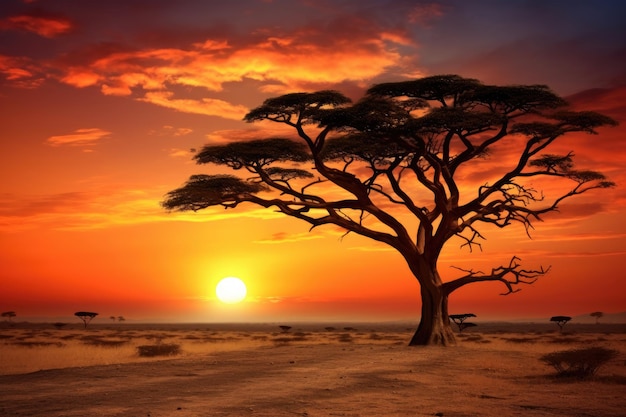This image captures a serene, almost cinematic scene reminiscent of an African savanna at sunset, evoking moments from The Lion King and Black Panther. In the distance, the sun is setting, casting a red, orange, and purple hue across the sky, particularly vivid in the top right corner. The landscape below is a sandy or yellowish ground interspersed with tufts of yellow grass and scattered plants. Dominating the scene is a large, distinct tree with bare branches at the base and a lush canopy of leaves concentrated on the upper right side. Near the tree, an animal is faintly visible, adding life to the tranquil setting. The overall ambiance is calm and evocative, capturing the raw beauty of nature.